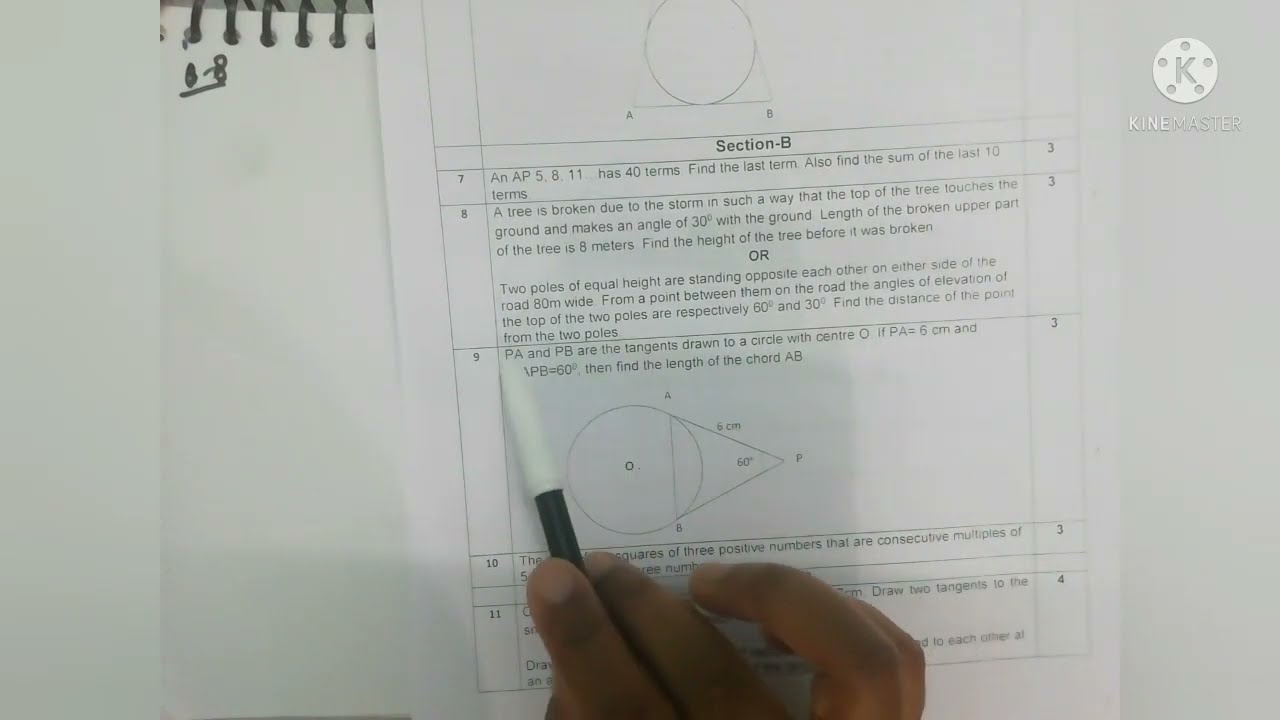The image showcases a vertical, rectangular frame of a light gray or white background. At the center, a sheet of paper with various math and geometry problems is placed on top of a black spiral-bound notepad. The sheet prominently features a heading that reads "Section B." Visible math problems include numbered questions and figures such as circles and triangles, along with labels like points A, B, and C on a triangle. Instructions within the problems mention tasks such as finding the last item, the sum of the last 10 terms, and a scenario involving a tree broken in a storm, forming a 30-degree angle with the ground, with an 8-meter-long broken upper part, requiring the calculation of the tree’s original height. The hand of an individual, emerging from the bottom center of the image, holds a black marker with a white tip, positioned as if pointing to the problems. A logo is visible at the upper right corner of the paper, contributing to a classroom-like setting with colors dominated by black, white, gray, and hints of brown.